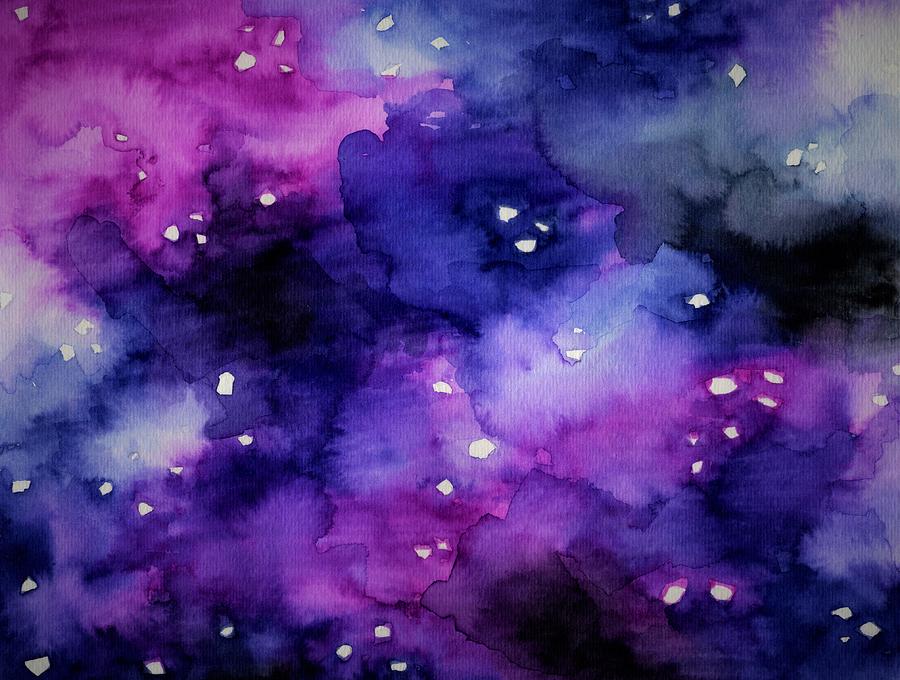This rectangular image, slightly wider than it is tall, resembles an abstract watercolor painting, evoking the essence of a galaxy or a sunset sky. Dominated by a harmonious blend of blacks, purples, pinks, blues, grays, and whites, the colors create a fluid, splotched composition with intricate ridges where the pigments bleed into each other. The top right and bottom sections feature prominent pink hues, while the bottom area is enveloped in darker tones, giving it a somber yet captivating depth. Scattered throughout the painting are small, white, cloud-like shapes that seem as if chunks were meticulously cut out, adding a layer of complexity and highlighting the star-like details in the abstract representation of the sky. Despite its abstraction, the image conjures a mesmerizing vision of the cosmos, where colors seamlessly merge to form an immersive, celestial artwork.